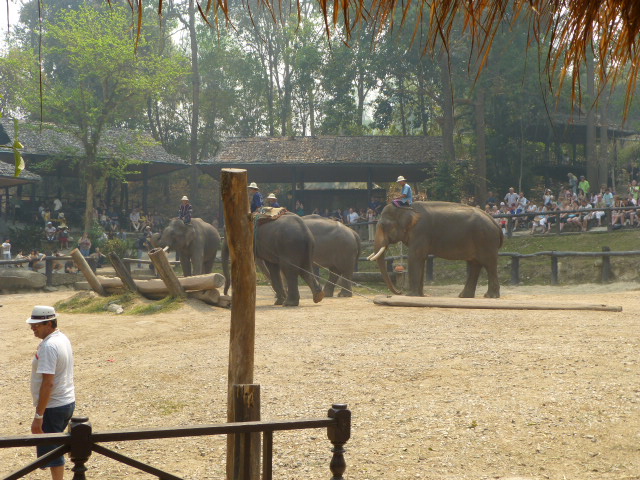The photograph captures an outdoor event featuring an open, yet roofed, structure with multiple seating areas where spectators are watching the scene below. In the center of the image, there are four Indian elephants on a dirt or gravel field. Each elephant is ridden by a person in tan safari hats. One of the elephants is dragging a large log with two ropes extending from its front. The field is enclosed by several rows of log-style fencing and surrounded by a crowd of onlookers, suggesting a zoo or wild animal park setting. In the foreground, on the left, a man in a white fedora-styled straw hat, white polo shirt, long black shorts, and what appears to be a white watch on his left arm stands behind a wrought iron gate and wooden post. The enclosure also features a wooden structure for storing large logs, with some grass growing around its base. The background is dotted with trees and large buildings with palapa-like roofs, enhancing the theme of an exotic, wildlife-centric event.